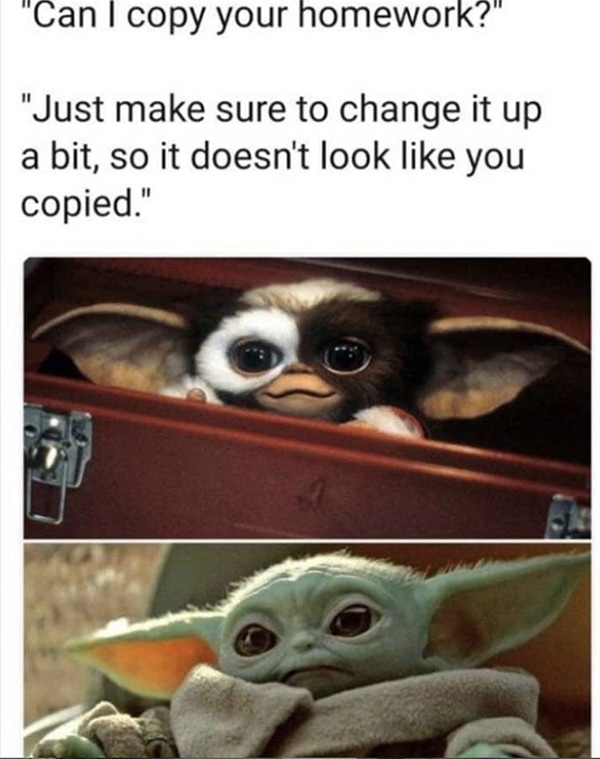This meme features a humorous comparison between two iconic creatures from popular culture. The top half of the image shows a small gremlin-like creature with very large ears, big brown eyes, and white and brown hair on its face, emerging from an open brown suitcase with silver clasps. The bottom half of the image directly below the gremlin shows Baby Yoda, also known as Grogu, with similar huge ears and brown eyes but in a pale green color. Baby Yoda is wearing a coat and has a contemplative expression on his face, mimicking his usual wise demeanor. The background details are not clear. Overlaying the images, there is text at the top that humorously reads, "Can I copy your homework? Just make sure to change it up a bit so it doesn’t look like you copied." The meme utilizes colors like white, black, brown, tan, green, orange, and yellow, and emphasizes the striking yet funny similarities between the two characters, despite their differences in color and expression.